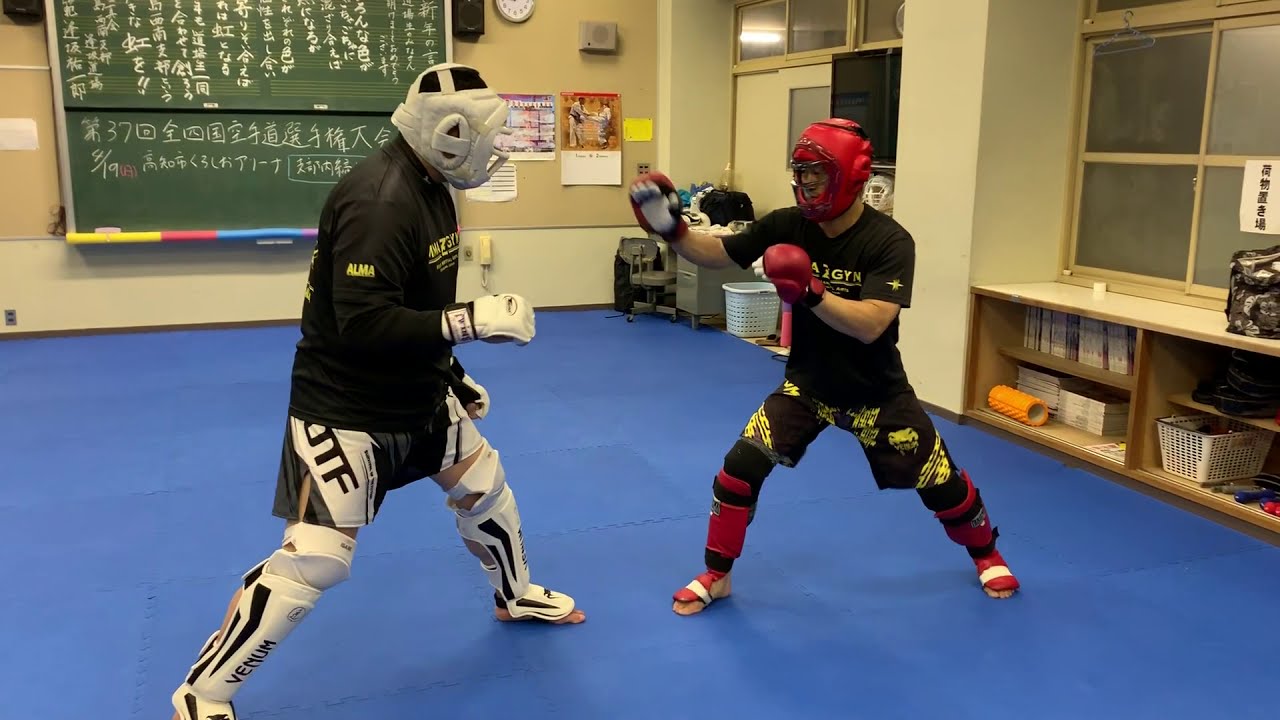This photograph captures an intense moment between two men engaged in a martial arts match, possibly boxing or kickboxing, in what appears to be a martial arts school. The indoor setting features beige walls and a blue floor comprised of interlocking foam squares. On the left of the image, one man is shown in profile, wearing a black tunic over white and black leggings, protective shin guards with black and white graphics, white gloves, and a white helmet. His right arm is slightly bent and extended toward his opponent. On the right side of the image, his opponent faces slightly forward in a three-quarter profile, clad in a black tunic with white writing, black and white shorts over black and red leggings with red protective padding, and red gloves. This man’s forearms are bare, and he wears a red helmet with a caged faceguard. He is in a lunging stance, with his right leg forward and left leg back, preparing for action. The background features a beige wall with a green chalkboard covered in Asian writing, likely Chinese characters, and a doorway leading to a hallway. To the right, there is a square-paned window above shelves filled with books and files. The setting is devoid of spectators, emphasizing the focused and disciplined environment of the martial arts school.